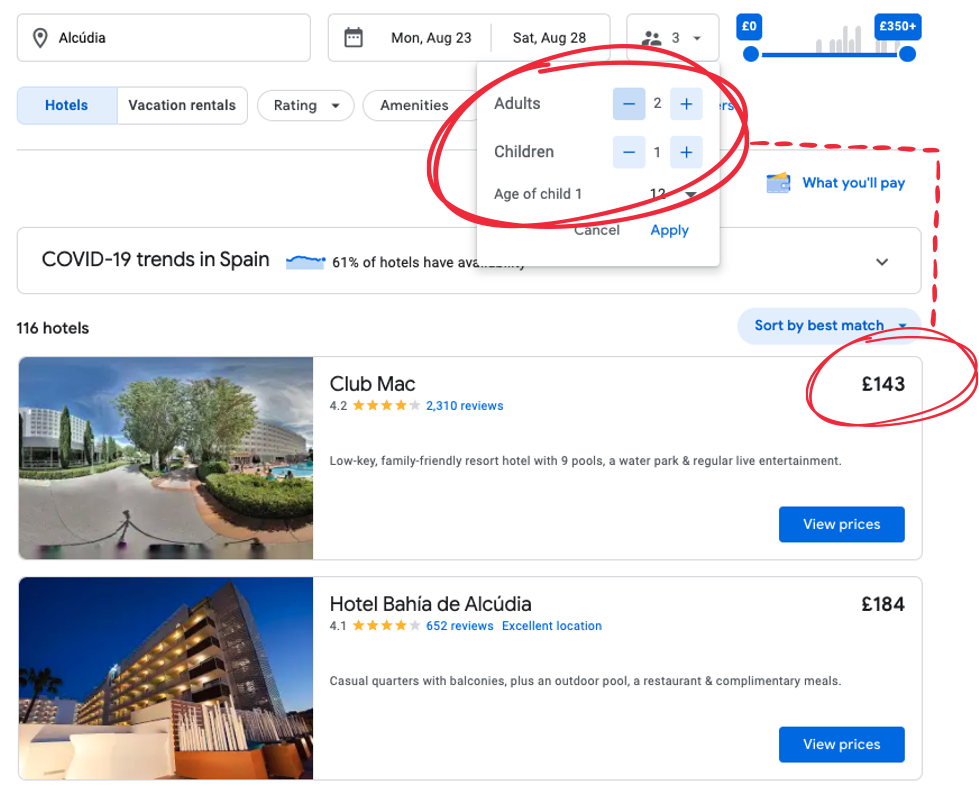**Caption:**
A snapshot of a hotel website for accommodations in Al-Qudiyah, showcasing an upcoming stay from Monday, August 23rd to Saturday, August 28th for two adults and one child aged 12, highlighted in red. Below this, there is information about COVID-19 trends in Spain, slightly obscured, indicating 61% hotel occupancy. Additionally, there's a calculator tool available to estimate the trip's cost, along with options for vacation rentals, ratings, amenities, and sorting preferences. The site lists 116 hotels, currently sorted by best match, featuring:

1. **Club Mac**: A family-friendly resort with a rating of 4 stars from 2,310 reviews. It offers nine pools, a water park, and live entertainment. Pricing, circled in red, starts at 143 euros. A picture of the hotel, along with detailed pricing information, is provided.

2. **Hotel Bia de Alcudia**: Priced at 184 euros, this hotel offers casual quarters with balconies, an outdoor pool, a restaurant, and complimentary meals. A picture of the hotel and a link for more pricing details are available.